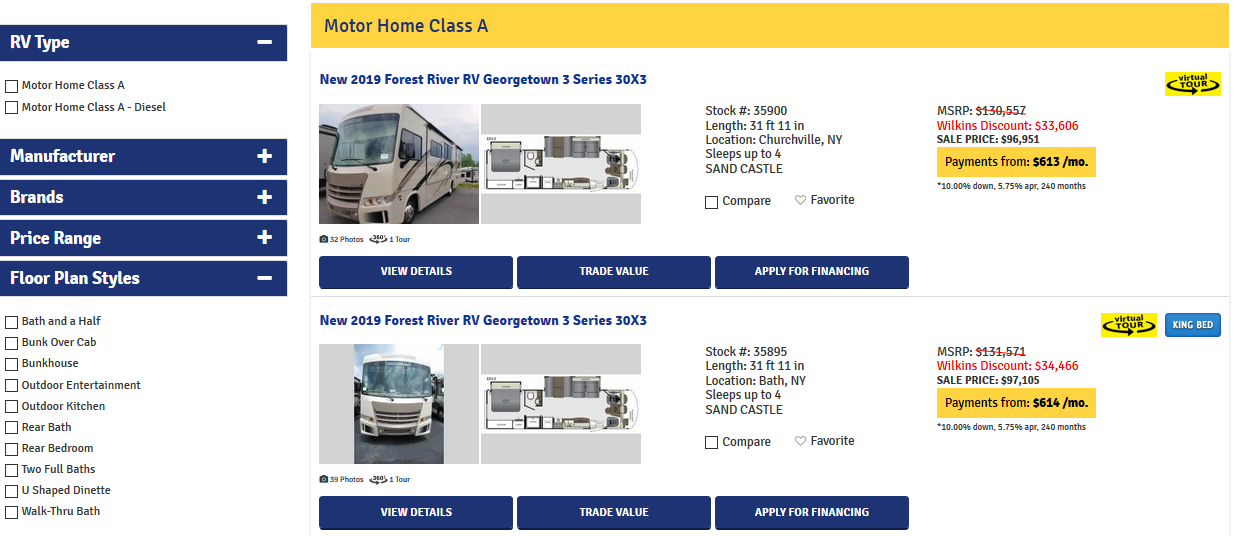This screenshot captures the shopping page of a website designed for browsing recreational vehicles (RVs). 

**Left Sidebar:**  
The sidebar, situated on the left side of the page, features a white background with dark blue tabs adorned with white text. The top tab reads "RV Type" and has a white minus sign on its right, indicating it is expanded. Below this tab are two checkboxes labeled "Motorhome Class A" and "Motorhome Class A-Diesel." Further down, the sidebar displays four additional tabs with plus signs next to them, signifying expandable sections: "Manufacturer," "Brands," "Price Range," and "Floor Plan Styles." The "Floor Plan Styles" tab is expanded, revealing a list of options with checkmarks beside each item on a white background. The listed styles include:  
- Bath and a Half
- Bunk Over Cab
- Bunk House
- Outdoor Entertainment
- Outdoor Kitchen
- Rear Bath
- Rear Bedroom
- Two Full Baths
- U-Shaped Dinette
- Walk-Through Bath

**Main Content Area:**  
To the right of the sidebar is the primary section of the website, characterized by a white background and a yellow header. The header features dark blue text that reads "Motorhome Class A." Below the header, two RV listings are presented in a similar format.

**First Listing:**  
- **Title:** New 2019 Forest River RV Georgetown 3 Series 30X3 (in blue text, positioned at the top left)
- **Image:** A front-left angled exterior view of the RV, featuring a beige or gray color scheme
- **Floor Plan:** A simplistic overhead view of the RV’s interior layout, situated to the right of the exterior image
- **Details:** Text-based information about the RV, positioned to the right of the floor plan

**Second Listing:**  
- **Title:** New 2019 Forest River RV Georgetown 3 Series 30X3 (similarly labeled as the first)
- **Image:** A front-facing exterior view of the RV
- **Floor Plan:** An almost identical overhead view of the RV’s floor plan located to the right of the exterior image
- **Details:** Additional information about the RV, similarly situated to the right of the floor plan

This detailed description provides a comprehensive overview of the shopping page’s layout and the content it offers to potential RV shoppers.